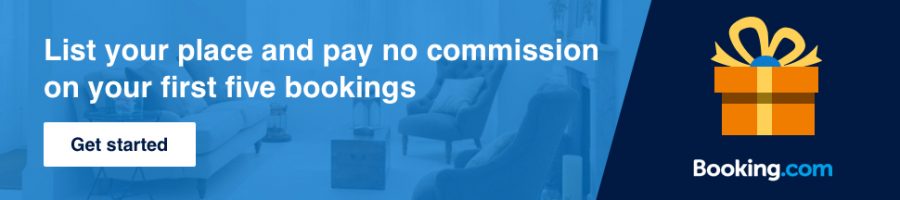This advertisement is designed as a web banner, potentially used in Google Ad programs or as an independent ad, promoting Bookings.com. The banner features a split background, with the left side in a light blue hue and showcasing a cozy living room setup. This setup includes a couch, two chairs, and a central table or box, emulating a homely and inviting atmosphere.

On the left side, the white text reads: "List your place and pay no commissions on your first five bookings." Beneath this text, there's a white rectangular button with the prompt "Get Started" in blue font, inviting potential customers to take action.

The right side of the banner shifts to a dark blue background. Here, an icon of an orange present, adorned with a slightly lighter orange ribbon, bow, and a blue dot on top, adds a touch of visually appealing contrast. Below this icon, "Bookings.com" is displayed prominently, with "Bookings" in white and “.com” in blue, maintaining the brand’s recognizable color scheme. The dark blue side features no other elements, allowing the message and call to action on the left to stand out distinctly.